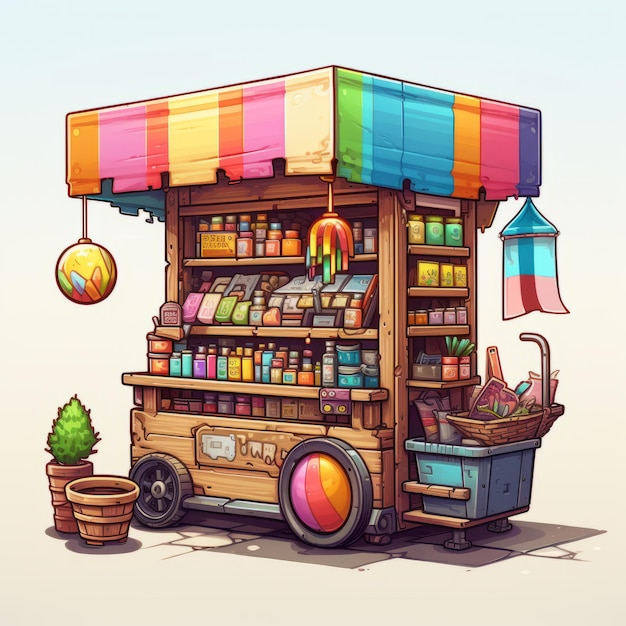This vibrant artwork is a color illustration of a large wooden vendor's cart, approximately nine feet tall. The cart is depicted in a three-quarter view, showcasing one side and one end. It features four shelves filled with a variety of colorful bottles and jars, arranged neatly across the structure. The cart is mounted on four wheels, with the front wheel nearest to the viewer being notably larger and adorned with pink, red, and orange stripes, while the smaller back wheel has six spokes.

A prominent feature of the cart is its rainbow-colored curtain canopy, which sports vibrant stripes in shades including orange, pink, red, yellow, green, blue, and purple. The canopy is embellished with various ornaments hanging from its corners, such as lanterns, spheres, ribbons, and flags. On the right end of the cart, a shelf protrudes outward, holding a bluish-green basket filled with items that appear to be food or herbs.

In the bottom left corner of the image, two wooden pots rest on the ground. One pot is narrow and taller, containing a green plant, while the other is shorter and wider. This detailed and colorful depiction underscores the cheerful and lively nature of the scene, likely representing a bustling marketplace or a whimsical vendor's stand.